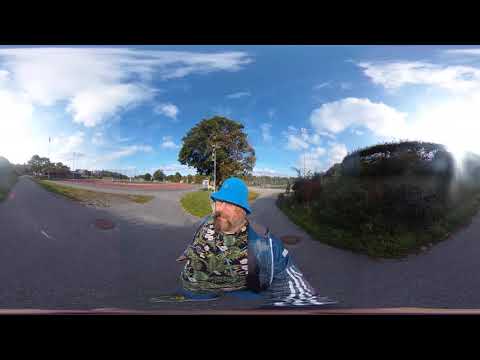This horizontally-aligned rectangular photograph, framed with thick black borders at the top and bottom, showcases a serene outdoor scene under a bright blue sky adorned with wispy white clouds. Dominating the middle ground sits a grassy patch with a solitary tree, surrounded by roadways extending into the distance on either side. Distant trees forge a verdant backdrop that frames the entire scene. A large, older white man stands in the foreground, his upper body emerging from the road's distorted perspective, possibly created by a fisheye lens effect. This distortion causes the road lines to seemingly merge into his brightly colored attire, which includes a green and black patterned shirt, a blue and green jacket, and a striking blue bucket hat. His gray and brown beard and partially obscured face due to the hat's brim add to the unique visual impact of this vibrant, sunlit photograph.